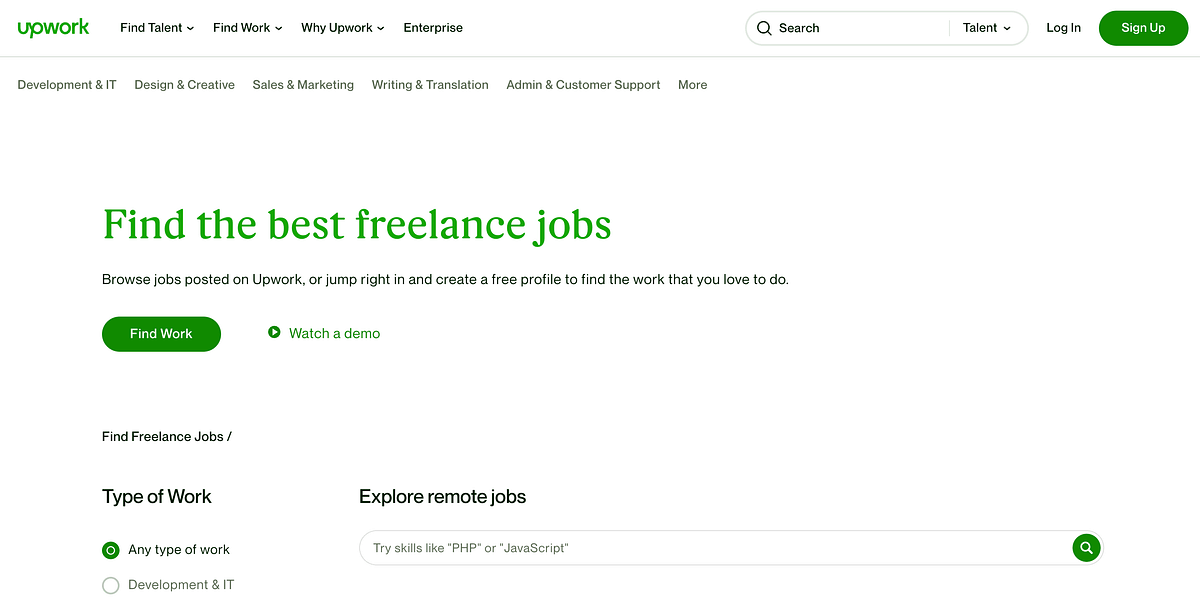The image features the Upwork website interface. In the top-left corner, the Upwork logo is displayed in green text. To the right, there is a horizontal menu with options: "Find Talent," "Find Work," "Why Upwork," and an "All" category, each accompanied by a drop-down arrow for further selection. Additionally, the word "Enterprise" is shown in black text. 

Underneath this menu, a search box labeled "Talent" with a drop-down function is depicted. To its right, there's a "Login" button in black text. Further to the right, a prominent green "Sign Up" button is displayed with white text. A long horizontal gray line spans the width below these elements, segmenting the upper navigation from the rest of the content.

In the center of the image, large green text reads, "Find the Best Freelance Jobs." Smaller black text below it encourages visitors to "Browse Jobs Posted on Upwork, or jump right in and create a free profile to find the work that you love to do."

Near the bottom-left corner, there is a green button labeled "Find Work." Next to it, a green play icon points to the right with accompanying text that says, "Watch a Demo" in green. At the extreme lower left, a selection bubble indicates "Any Type of Work" with a green dot signifying that this option is currently selected.